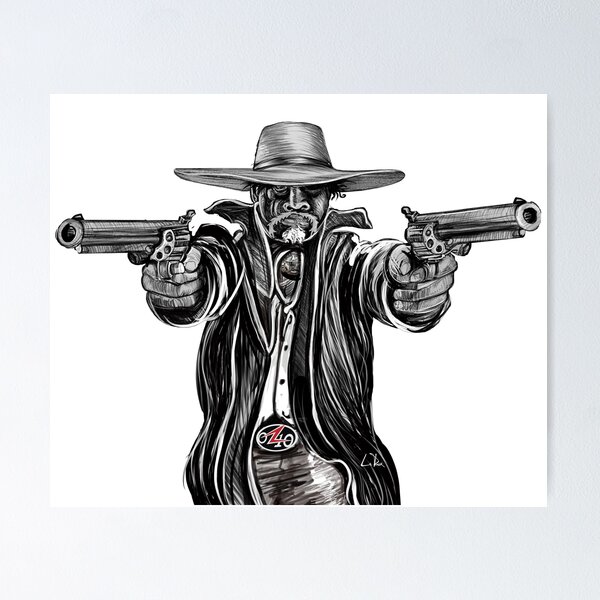The image is a square and artistically drawn in a predominantly black and white color scheme with a few colored elements. It features a light gray background, perhaps suggesting a wall, with a centrally placed large white square poster. This poster displays a detailed sketched image of a cowboy facing directly towards the viewer. The cowboy sports a wide-brimmed hat that casts a shadow over his eyes, giving him a fierce look. His face is adorned with a graying goatee. The cowboy is clad in a long black jacket over a white shirt, and though partially obscured, he appears to be wearing blue jeans.

Prominently displayed in front of him are two drawn revolvers, their barrels visible. His belt buckle is notably large and inscribed with the numbers "0 4 0" or "0 Z 0", where the character in the middle is a vivid red, standing out as the only colored element in the belt buckle. The image is framed by a blue border, thicker at the top and bottom than at the sides, though nearly washed out on the left side.